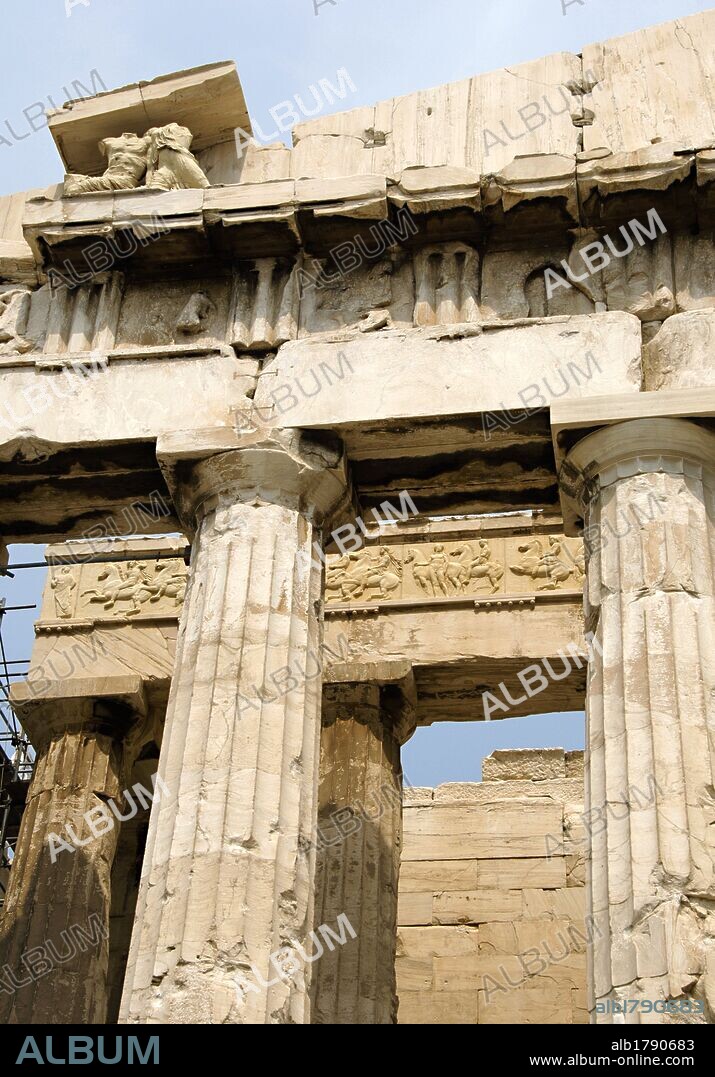The image appears to be from a website, as indicated by a black bar at the bottom that reads "album" on the left and has the text "ALB 1790683 www.albumonline.com" on the right. Additionally, the word "album" appears diagonally in light white text as a watermark across the image. The scene depicts an ancient archaeological site, possibly from Rome or Greece, featuring old, weathered columns that are broken in places. Two prominent columns with straight vertical lines are in the foreground, holding up a crumbling structure adorned with carvings. The carvings include intricate artistic drawings, some depicting men riding horses. Behind this main structure, there are more columns and large stacked stone or cement blocks, hinting at further ruins and larger stone walls in the background. Above the columns, there are artistic representations, possibly two figures that look like dogs or demons, with a glimpse of blue sky beyond the ancient remains.